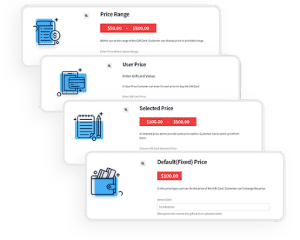In this image, there are four cascading boxes arranged diagonally from the upper left to the lower right. Each box features a small, indiscernible blue symbol on the far left side. Within these boxes, three contain smaller red boxes, though the text inside these red boxes is too small to be easily read. The boxes are topped with bold black headings: "Price Range," "User Price," "Selected Price," and "Default Fixed Price," respectively. Below these headings, there is additional text, but it, too, is difficult to decipher due to its small size. Each box is surrounded by a thin gray border, adding definition to their shapes. Additionally, there is an 'X' icon on the left side of each heading, likely indicating a close or delete function for the boxes.